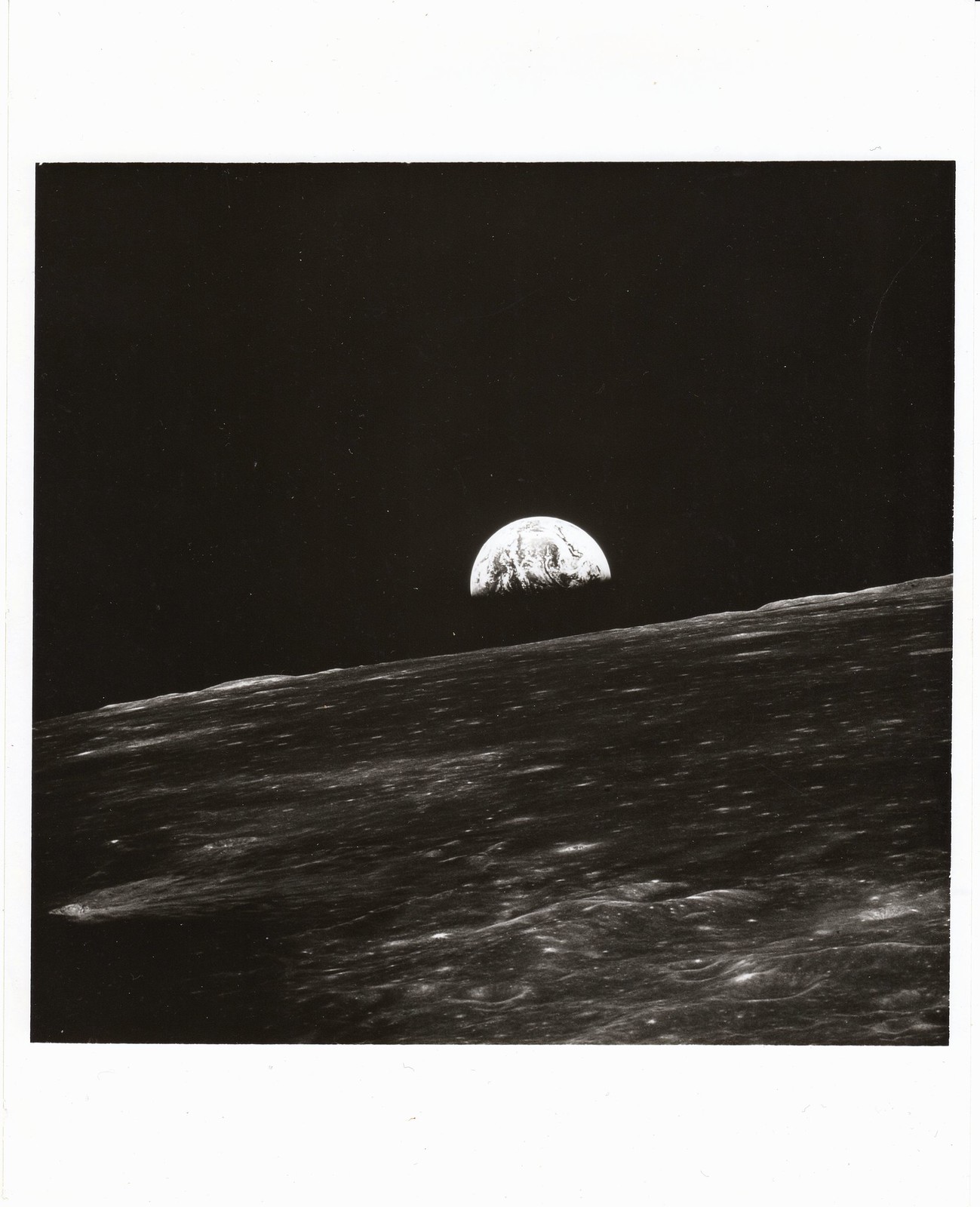The image is a black-and-white photograph, seemingly taken from outer space. Dominating the top half of the picture is a bright half-moon against a black sky, detailed with dark lines from craters and other surface features. The moon appears at a slight 30-degree tilt to the left. The bottom half of the image, ambiguously gray and white, suggests surface features—possibly Earth's surface with faint lights and cloud patterns, although this is not clearly distinguishable. The overall composition suggests the perspective of a photograph taken from a spacecraft, perhaps showing an Earthrise or Moon-set, with scattered stars visible against the dark background. The extreme darkness of the image makes finer details difficult to discern.